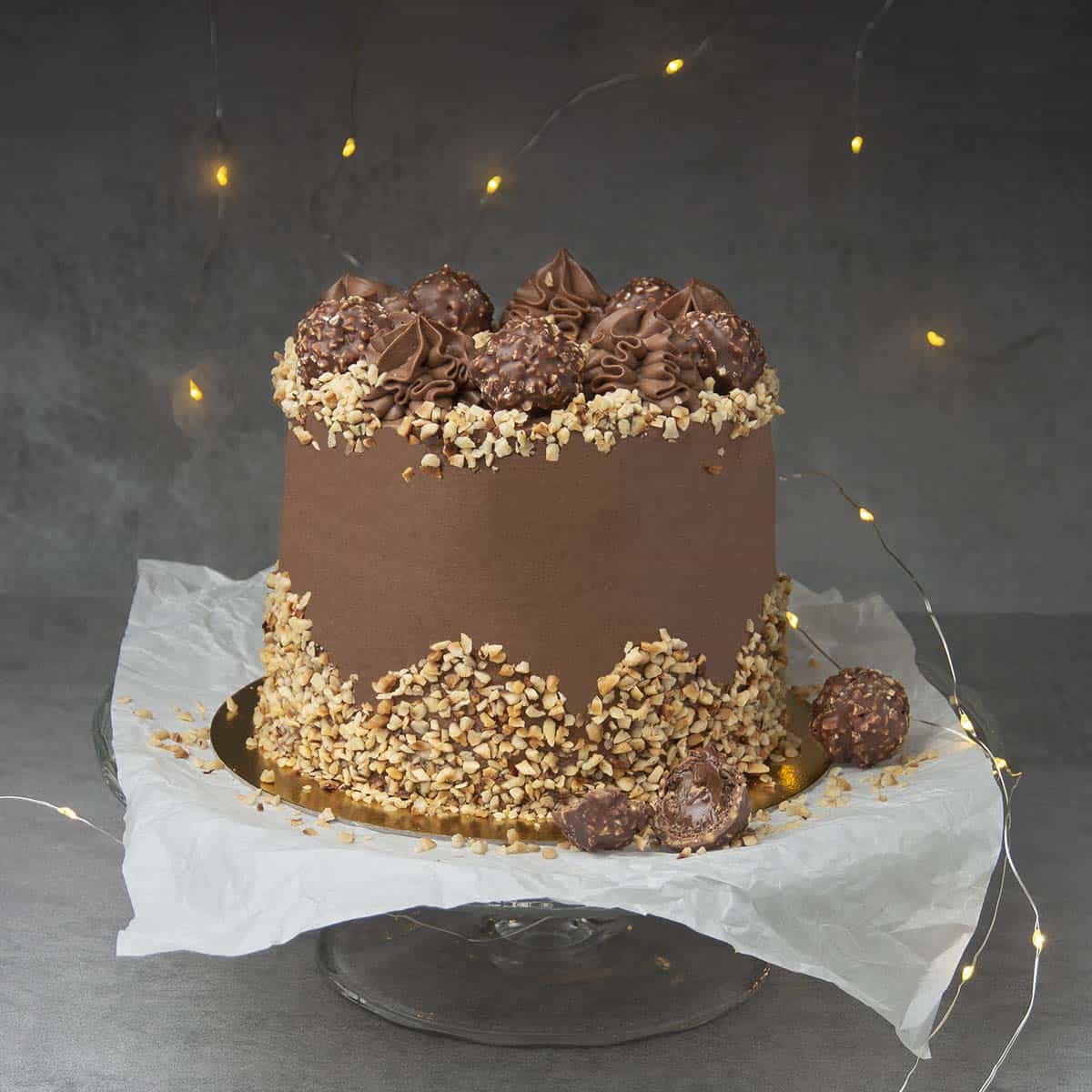This detailed photograph features a tall, cylindrical chocolate cake with a smooth, dark brown frosted exterior. The cake is embellished with chopped cashews and nuts, which are lighter brown in color, adorning both its base and top. At the top, intricate designs resembling chocolate flowers have been piped using dark brown cream, adding a touch of elegance. Additionally, there are a couple of chocolate truffles positioned at the top and two more near the base of the cake. The cake rests on a round, clear glass cake stand, separated by a layer of white parchment paper. This stand is placed on a white-colored paper, contributing to the overall presentation. Surrounding the cake are a few threads or strands of Christmas-style fairy lights that emit a glowing yellow hue, set against a stark grey background, creating a festive and warm ambiance.